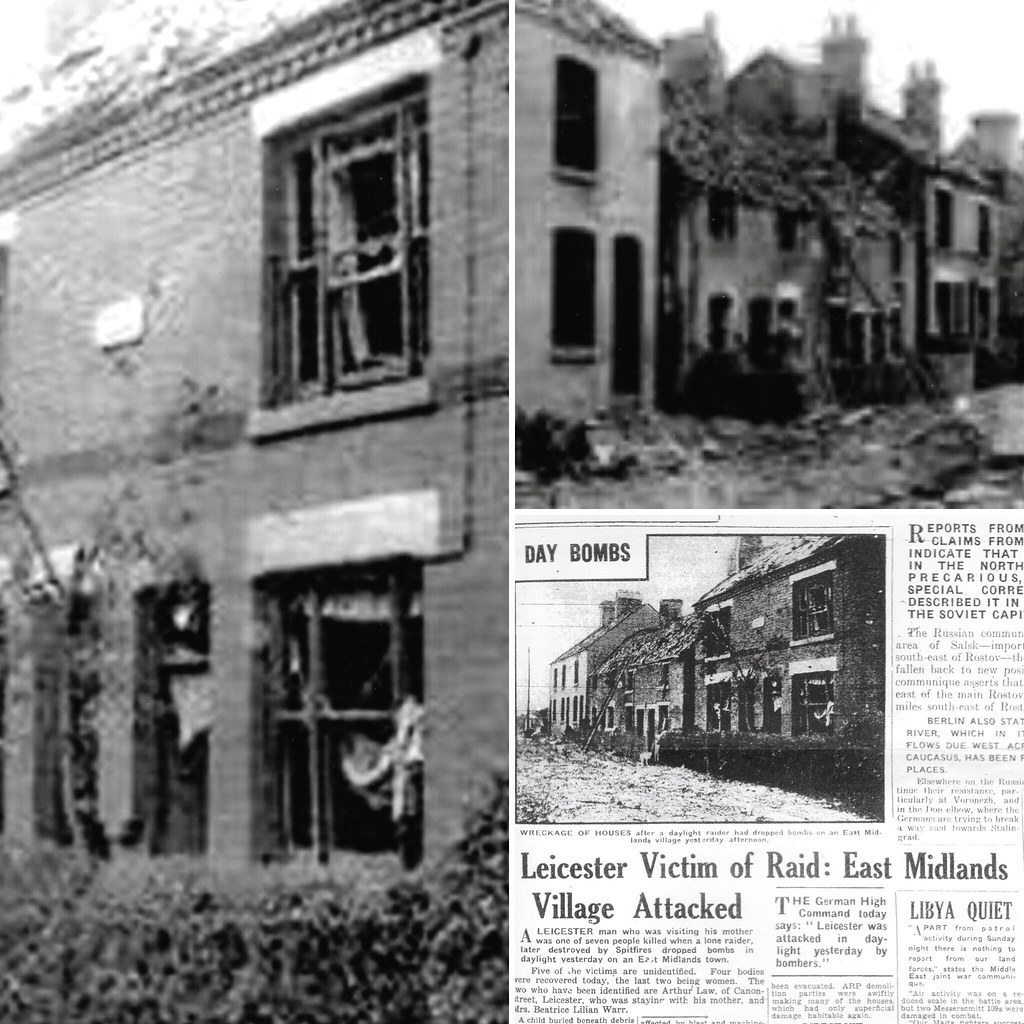The image appears to be an old black-and-white photograph of a newspaper page from what is likely World War II. The layout is relatively square and divided into three sections. On the left, we see an impactful close-up of a demolished building, with clear signs of intense damage such as broken windows and a severely damaged roof. The right side is split into two halves. On the top, there's a slightly less close-up black-and-white photograph showcasing more buildings that have been bombed, displaying significant devastation including caved-in walls and destroyed ground. Adjacent buildings on either side also show extensive ruin. Below this, the lower half contains an article titled "Day Bombs." Alongside the headline, "Leicester Victim of Raid, East Village Attacked," there's another image depicting more broken roofs and windows, suggesting widespread destruction. The article seems to report on the tragic events, likely caused by an air raid, and captures the stark reality of war-torn areas.